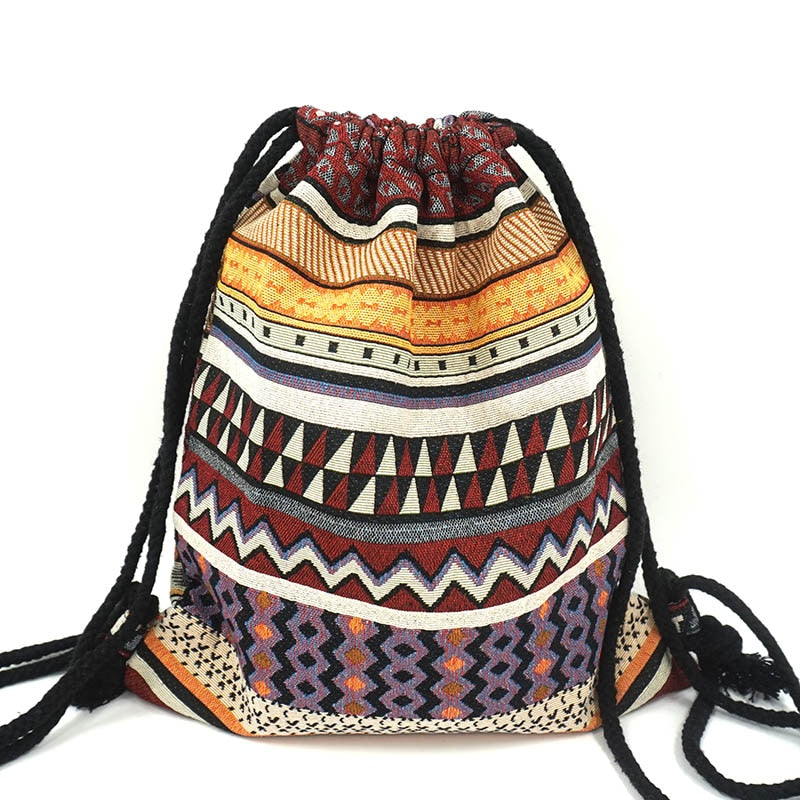The image depicts a drawstring-style bag boasting a vibrant and complex southwestern Native American-inspired design. The bag is adorned with an intricate array of geometric patterns and a muted yet rich color palette. Dominant hues include deep garnet red, maroon, yellow, orange, black, white, gray, and purple. The artwork features horizontal chevron stripes in red, stacked triangles in red and white, and solid lines in black, white, and cream—all interconnected to form a visually striking display. Notably, one stripe is dotted with black squares throughout its length. The top of the bag is characterized by yellow and orange stripes beneath a garnet red section, with more geometric patterns transitioning to chevrons and diamond shapes at the bottom in purple and dark shades. The bag's black woven yarn drawstrings are visible, coiled at the bottom and sides. The setting is a plain white background, highlighting the bag's detailed and eclectic design.